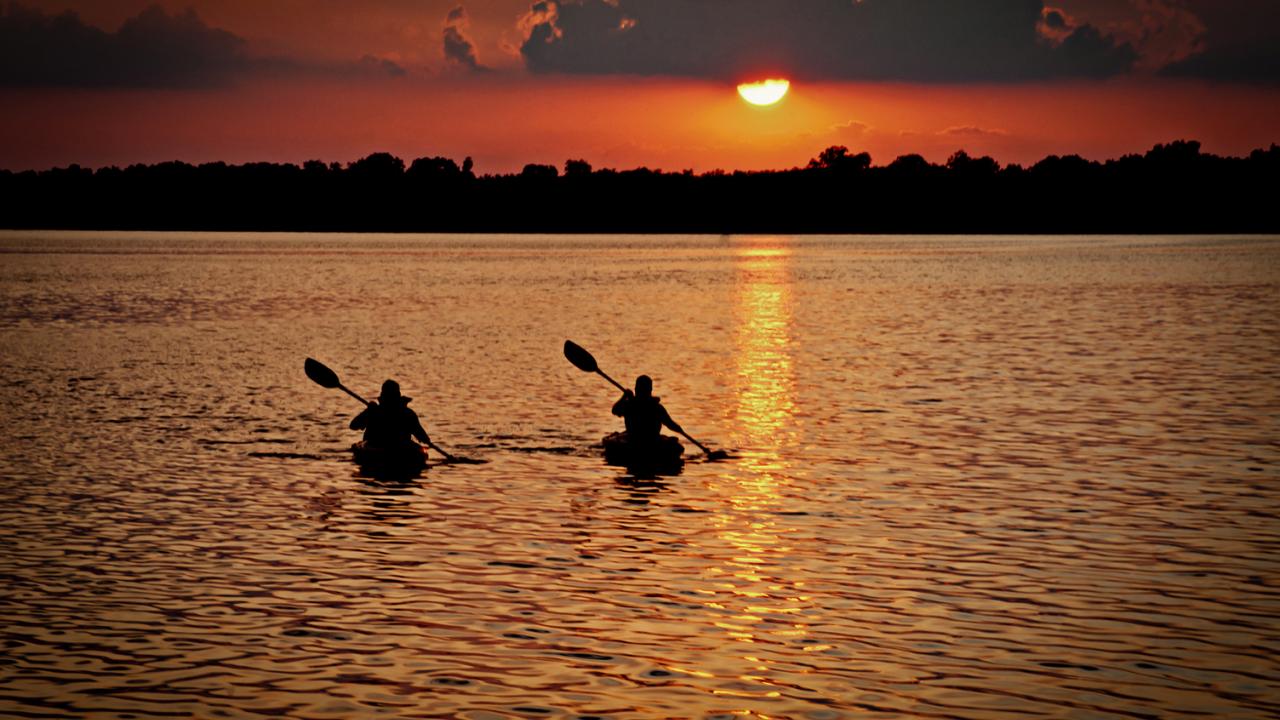The image captures a serene sunset scene over a vast body of water, likely the ocean. Dominating the foreground are silhouettes of two people in kayaks, paddling in unison. They are positioned on the left side of the center of the image, and their outlines are dark due to the shadow cast by the setting sun. Both have their oars submerged on the right side, creating a synchronized, dynamic effect. The sky above is a gradient of colors, transitioning from a deep blue with white clouds to a warm orange near the horizon. The sun, partially obscured by the clouds, is a striking orange hue and casts a glowing, reflective streak across the water’s surface, stretching from the foreground to the horizon. In the distance, the horizon is framed by a dark silhouette of trees and a faintly visible city skyline, adding depth to the scene. The overall clarity of the image is high, emphasizing the contrast between the dark kayaks and the vibrant sky. The water itself appears dark, likely contributing to the dramatic shadows enveloping the kayakers. This tranquil and picturesque setting beautifully captures the moment as day transitions into night.